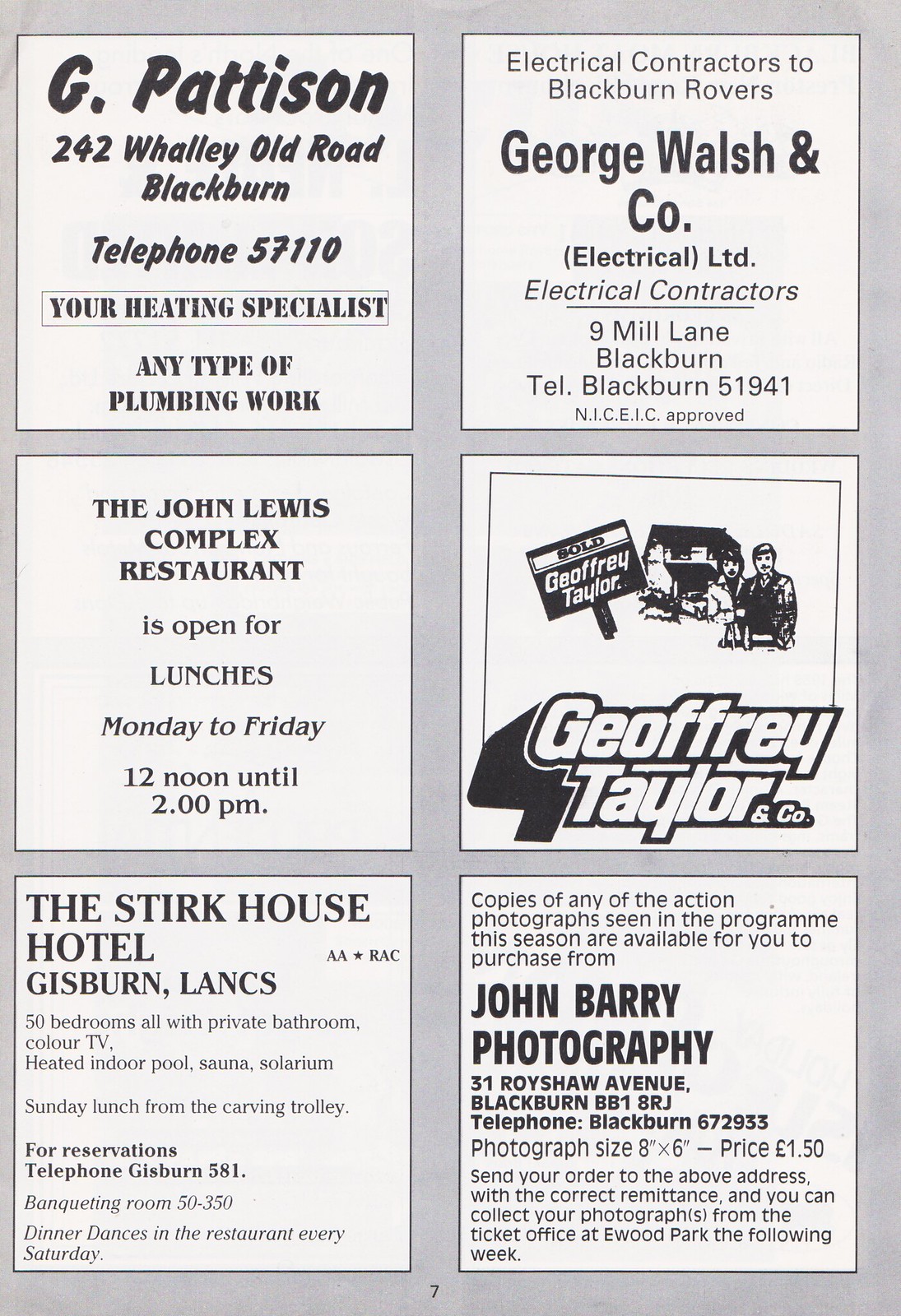The image appears to be a cutout from a newspaper or magazine featuring six distinct advertisements arranged in a grid against a light gray background, with outlined black squares, each containing white interiors. In the top left square, it reads: "G. Patterson, 242 Wally Old Road, Blackburn, Telephone 57110 - Your heating specialist, any type of plumbing work." Next to it, in the top right square, there's "Electrical Contractors to Blackburn Rovers, George Walsh & Co. Electrical Ltd, 9 Mill Lane, Blackburn, Tel: Blackburn 51941, NICIC Approved." 

In the middle left square, the advertisement states: "John Lewis Complex Restaurant is open for lunches, Monday to Friday from 12 noon until 2 p.m." The middle right square features "Jeffrey Taylor & Co. with a 'sold' sign and a black ink drawing depicting two people standing in front of a house." 

In the bottom left square, the ad for "Sturck House Hotel, Gisborne, LANCS" lists the amenities: "50 bedrooms all with private bathrooms, color TV, heated indoor pool, sauna, solarium, Sunday lunch from the carving trolley. Reservations Telephone: Gisborne 581. Banqueting Room capacity: 50 to 350. Dinner dances in the restaurant every Saturday." 

Finally, in the bottom right square, the ad for "John Barry Photography, 31 Walsh Avenue, Blackburn, BB1 8RJ, Telephone Blackburn 672933" mentions: "Copies of any action photographs seen in the program this season are available for purchase. Photographs size 8x6 inches, price $1.50. Send your order to the above address with the correct amount, and you can collect your photographs from the ticket office at Ewood Park the following week." The page is marked with the number 7 at the bottom, indicating its placement.